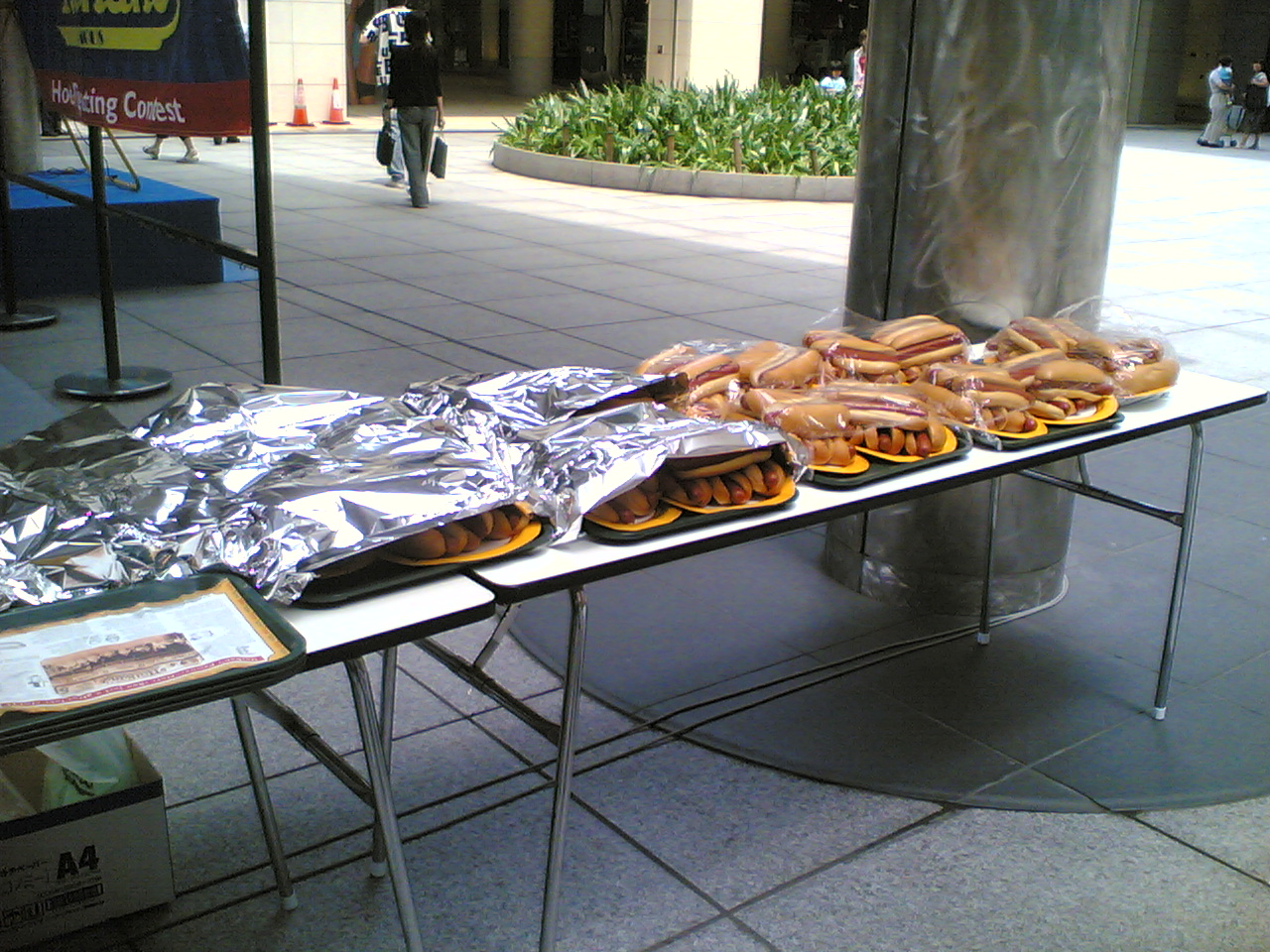This photograph captures an outdoor setting in a spacious plaza lined with cement pavers and various large buildings in the background. Central to the image are two long, white folding tables arranged diagonally across the frame. These tables are piled high with dozens of hot dogs in buns, meticulously arranged on yellow paper plates and placed atop rectangular gray trays. Some of the hot dogs are covered with clear plastic wrap, while others are wrapped in silver foil, creating a sense of preparation for a significant event. In the top left corner, a partially obscured sign reading "Hot Dog Eating Contest" hints at the occasion. The background features a circular planter brimming with lush green plants, people walking or sitting nearby, and occasional orange traffic cones adding to the bustling ambiance. A prominent silver post and temporary barriers further frame the scene, indicating a well-organized gathering.